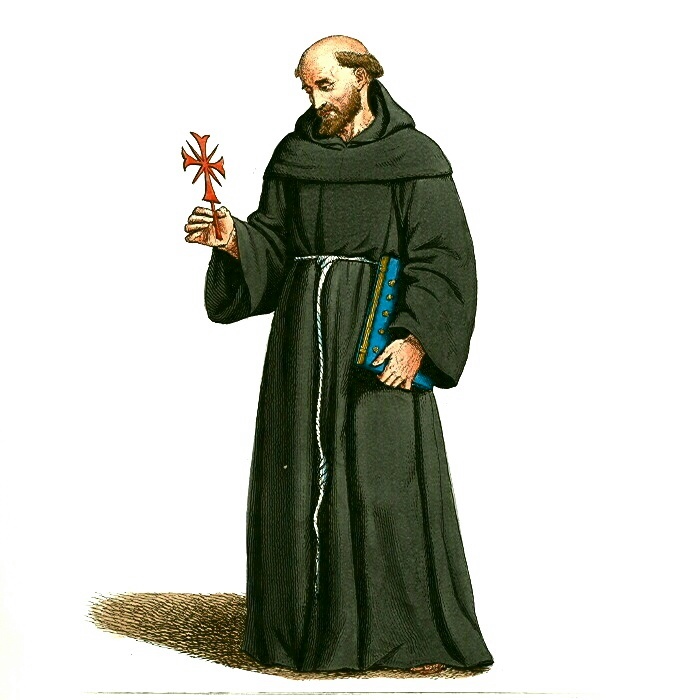This highly detailed, colored drawing depicts a thoughtful monk, identified by his traditional attire and contemplative expression. The monk has a bald head with brown hair framing the sides and back, complemented by a full beard. He wears a long, dark green robe cinched at the waist with a white rope belt, one end of which nearly reaches the ground. His right hand extends forward, clutching an orange cross adorned with two diagonal lines, while his gaze is directed downward at the cross, deep in contemplation. In his left arm, he cradles a large blue book with yellow trim, likely a Bible. The monk stands on a brown spot, with his shadow cast, suggesting he is in a well-lit area against a stark white background.